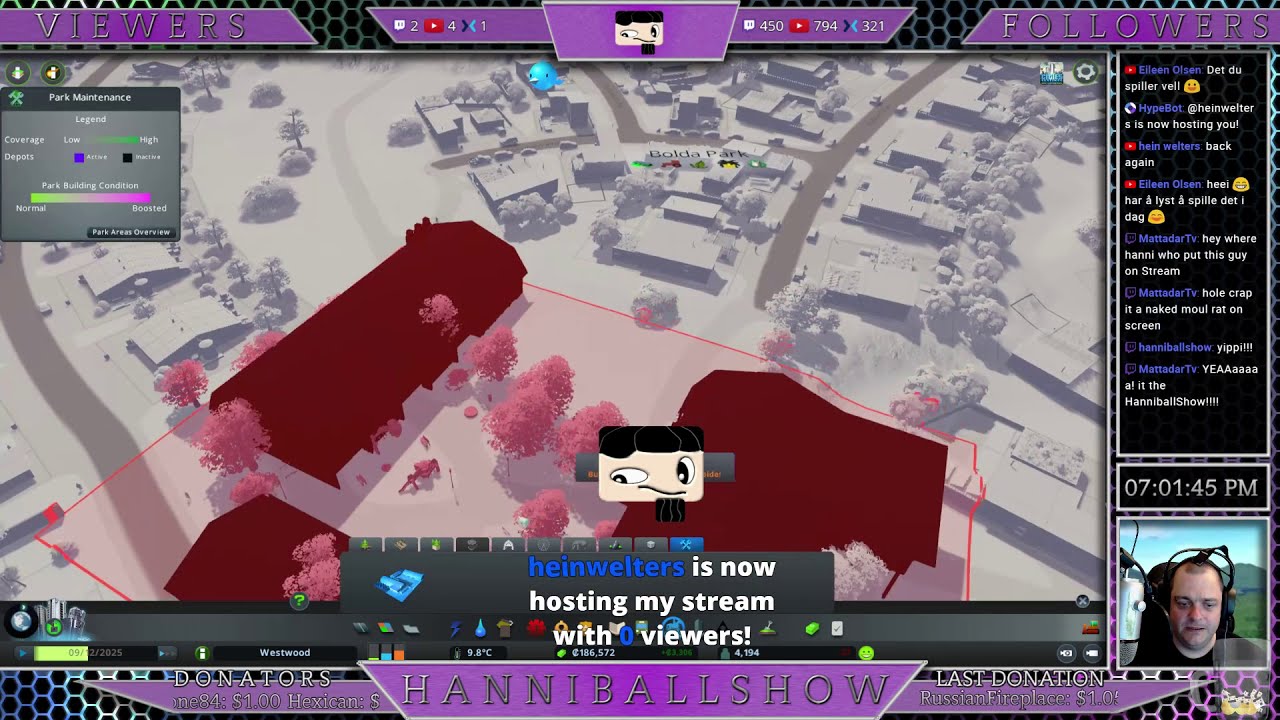This image is a detailed screenshot from a live stream, possibly a city-building game. The main image is surrounded by a purple and black border. In the center at the bottom of the screen, bold text reads "Hannibal Show," which likely indicates the streamer's username. The game itself shows an aerial view of some sort of cityscape or battle scene. In the bottom right corner, a camera feed displays the streamer—a white man with a shaven head, wearing a headset and positioned next to a microphone. Directly above the streamer is the time and a constantly updating chat window filled with messages from viewers. Additional text on the screen includes a notification, "Hein Walters is now hosting my stream with zero viewers," and various informational sections like followers and donators. The predominant colors in the image are purple, black, white, and shades of blue, grey, maroon, red, and pink.